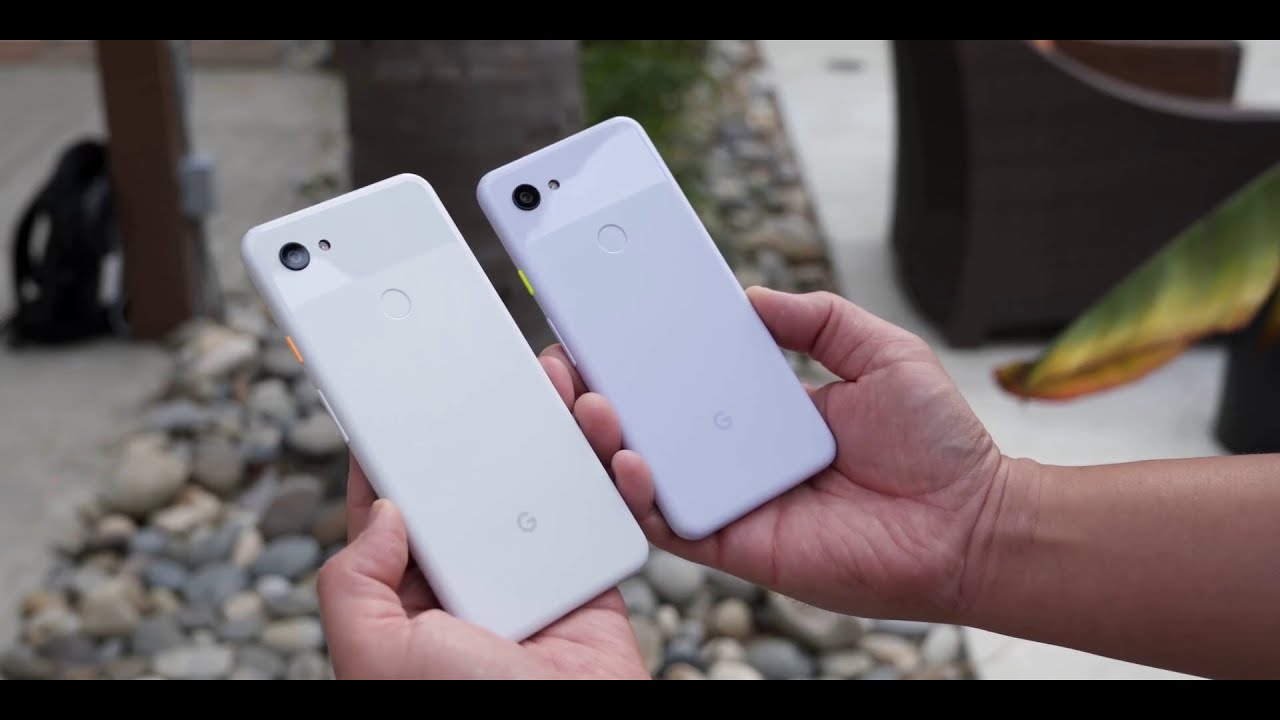In the foreground of this detailed image, a person with tannish white skin is holding two Google Pixel smartphones, each in the palm of their hand. Both phones share the signature Google 'G' logo on their bottom middle but differ slightly in color and size. The larger, pearly white phone rests in the left hand, juxtaposed with the smaller, ivory white phone in the right. No phone covers are attached to any of the devices, emphasizing their bare design. The background reveals a well-kept patio area adorned with rock landscaping and lush palm trees. On the left side, a brown pillar boasts a gray electric box and a black backpack leaning against it. Opposite, two large wicker armchairs nestle next to a vibrant green and yellow palm frond extending from a corner. The serene outdoor setting further contrasts with the detailed focus on the person comparing the two similar, yet distinct, smartphones.